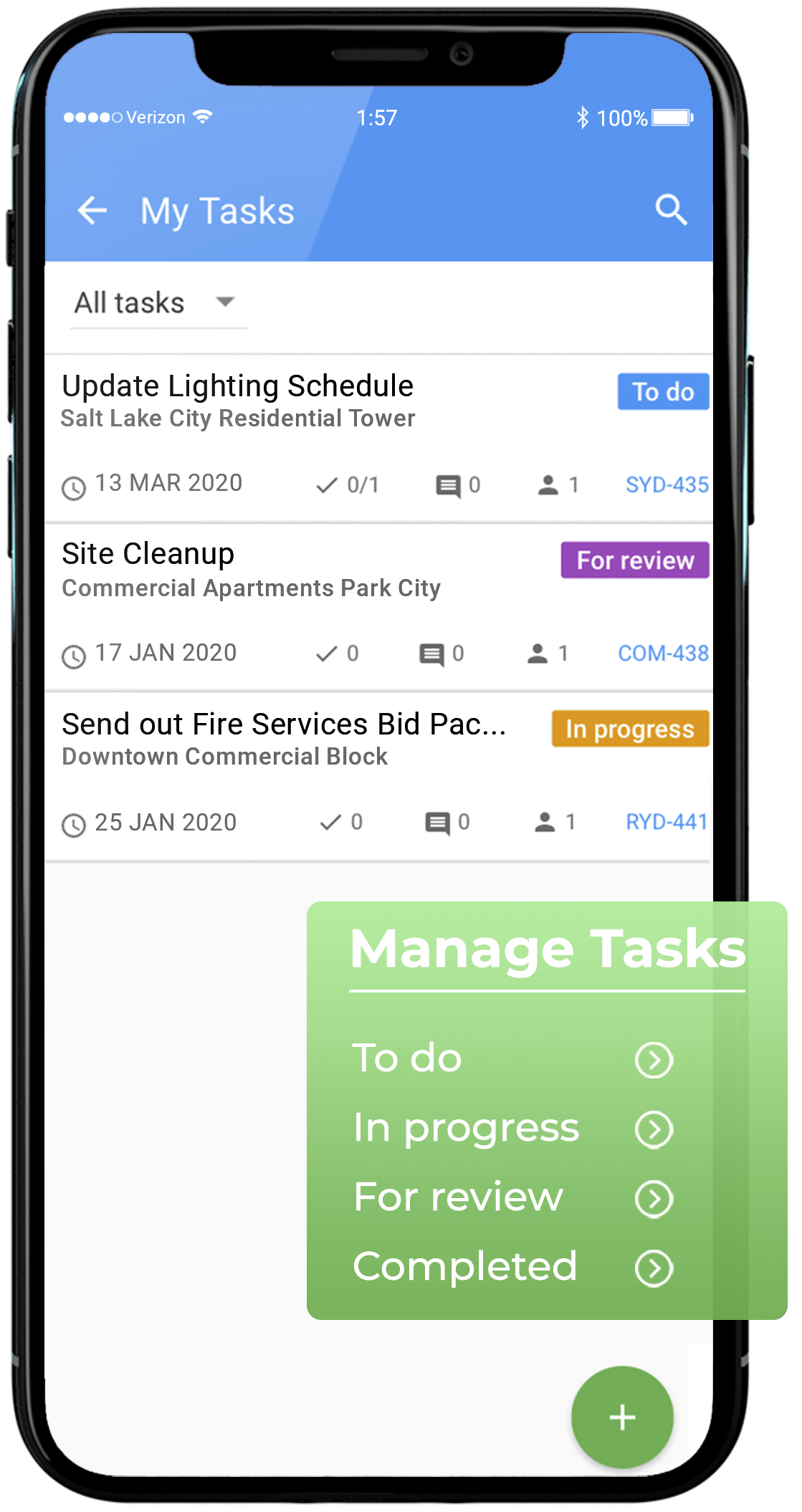The image showcases an iPhone screen displaying a mock-up of a task management website. The website interface, visible on the iPhone screen, prominently features a blue header titled "My Tasks." Below the header, there is a detailed list of three tasks, each accompanied by corresponding information.

The first task, "Update Lighting Schedule," is tagged with the location "Salt Lake City Residential Tower." Additional details include the date, March 13, 2020, a checkbox indicating zero out of one tasks completed, a speech bubble icon with a zero next to it, and a person icon with a one next to it. A colored box labeled "To Do" signifies the current status of this task.

The second task, "Site Cleanup," pertains to a commercial project located at "Commercial Apartments Park City." This task's status is marked as "For Review," using the same format as the first task.

The third task, "Send Out Fire Services Bid Pack," shows the location "Downtown Commercial Block." The text cuts off, ending in an ellipsis, and the task status is indicated as "In Progress."

Overlaying the iPhone screen is a green text box with the underlined title "Manage Tasks." Beneath this title is a list of different task statuses, including "To Do," "In Progress," "For Review," and "Completed," each accompanied by a right-facing arrow encircled as an icon.

This comprehensive layout provides a clear and organized view of ongoing tasks, their statuses, locations, and associated details, all within a user-friendly mobile interface.